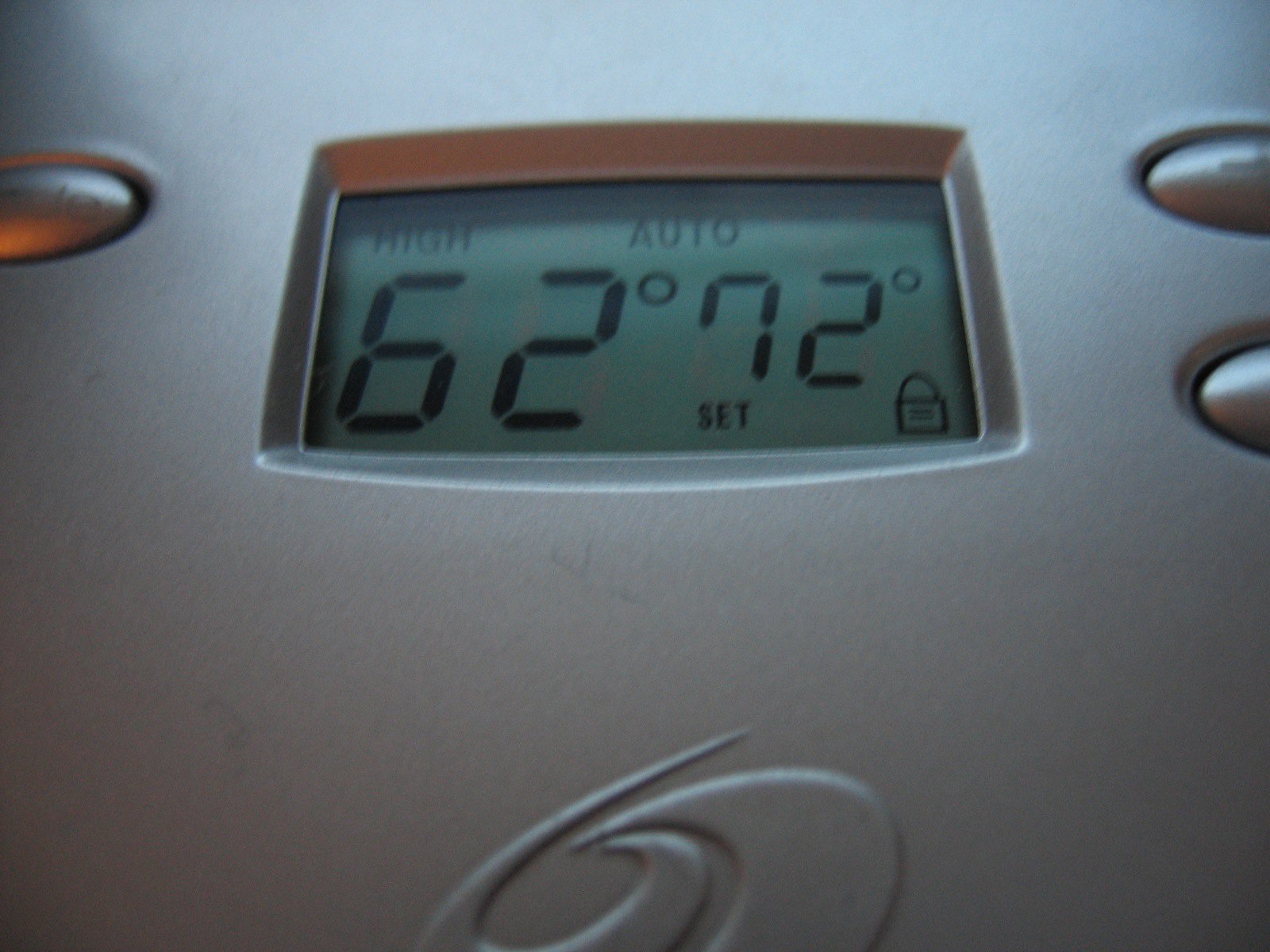The image features a metallic, shiny thermostat with a predominantly gray back. The device's surface includes a few distinctive details and indentations that resemble buttons. In the upper left corner, there's an indented area that blends with the overall color. Similarly, on the right side, two additional indentations are present, one partially visible in the upper right corner and another smaller one below it, both outlined to enhance visibility.

At the bottom of the panel, there's an engraved, wide, squiggly line. The centerpiece of the thermostat is a display window, covered with either clear plastic or glass, through which the settings are visible. The background of the display is a light gray, and the readings are shown in black text. To the left, the word "Hi" is displayed, and directly below it, a large "62°" indicates the current temperature setting. Following "Hi," to the right, the word "Auto" (A-U-T-O) is written, with another temperature reading of "72°." These readings include a small degree symbol next to each. At the bottom of the display, the word "Set" is present, and to the far right, there is a small diagram depicting a lock, the purpose of which is unspecified.